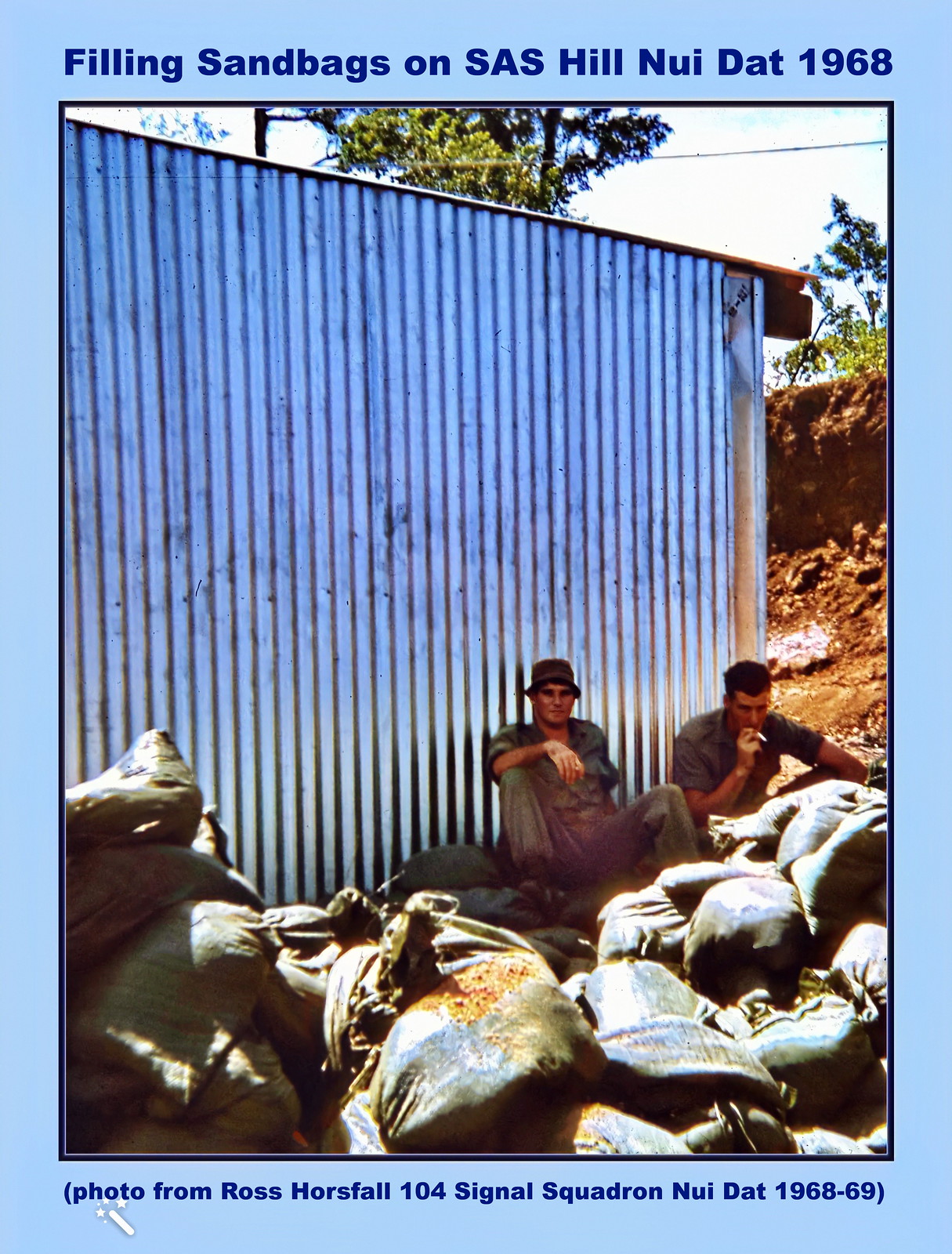The image is an old photograph taken in daylight, showcasing a scene from 1968. Under a clear blue sky, the image features a silver-colored shipping container surrounded by trees. Against the container sit two men in green uniforms, appearing weary; one smokes a cigarette. In front of them are numerous sandbags. The photograph has a light blue border and includes text at the top in blue lettering saying, "Filling sandbags on SAS Hill, Noidat 1968." Below the image, it reads, "Photo from Ross Horsfall, 104 Signal Squadron, Noidat 1968-69."